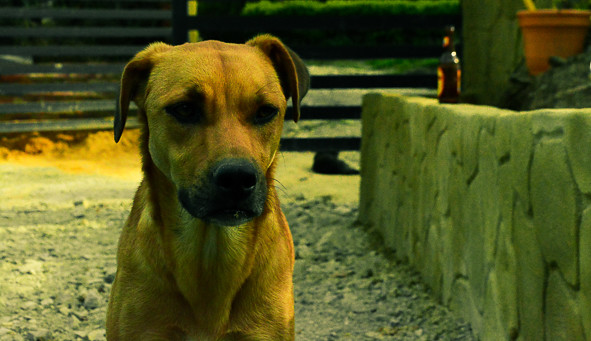The image captures a dog with short yellow-orange fur and a black nose and mouth, standing on a rough, earthy terrain scattered with rocks. The dog's breed is uncertain, resembling a mix between a golden retriever and possibly a yellow lab or Old Yeller, but distinct in its own way. Its black ears and somewhat darkly shaded mouth contrast with its bright coat. The dog's face and front body are in close-up, yet the illumination doesn’t clearly reveal its eyes. It appears healthy, fit, and strong, though it carries a slightly sad expression.

To the right of the dog is a stone wall, atop which rests a glass bottle resembling a bottle of beer. In the background, there’s a bench and, further to the right, a red plant pot. The setting is an outdoor enclosure with a dirt floor. There is also the presence of another animal seen sitting down within the enclosure.